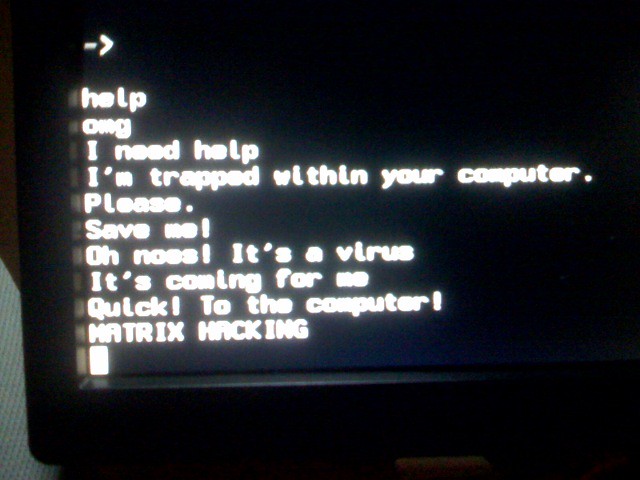This photograph captures a close-up of an old, black CRT monitor with a boxy design. The monitor's screen is mostly black, displaying a series of white text in lowercase and a few lines in all capital letters. At the top of the screen, there's a white arrow created with a hyphen and a greater-than sign. The text reads: "help OMG, I need help. I'm trapped within your computer. Please save me. Oh no, it's a virus. It's coming for me. Quick to the computer Matrix hacking." The phrase "Matrix hacking" is prominently displayed in all capital letters. Beneath this text, there's a small white square, likely representing a cursor. The background is dim and indistinct, with some visible gray fabric and possibly a brown floor, though the darkness of the photo makes further details hard to discern. The image overall feels blurry and out of focus, emphasizing the nostalgic feel of the scene, reminiscent of an old DOS prompt screen.